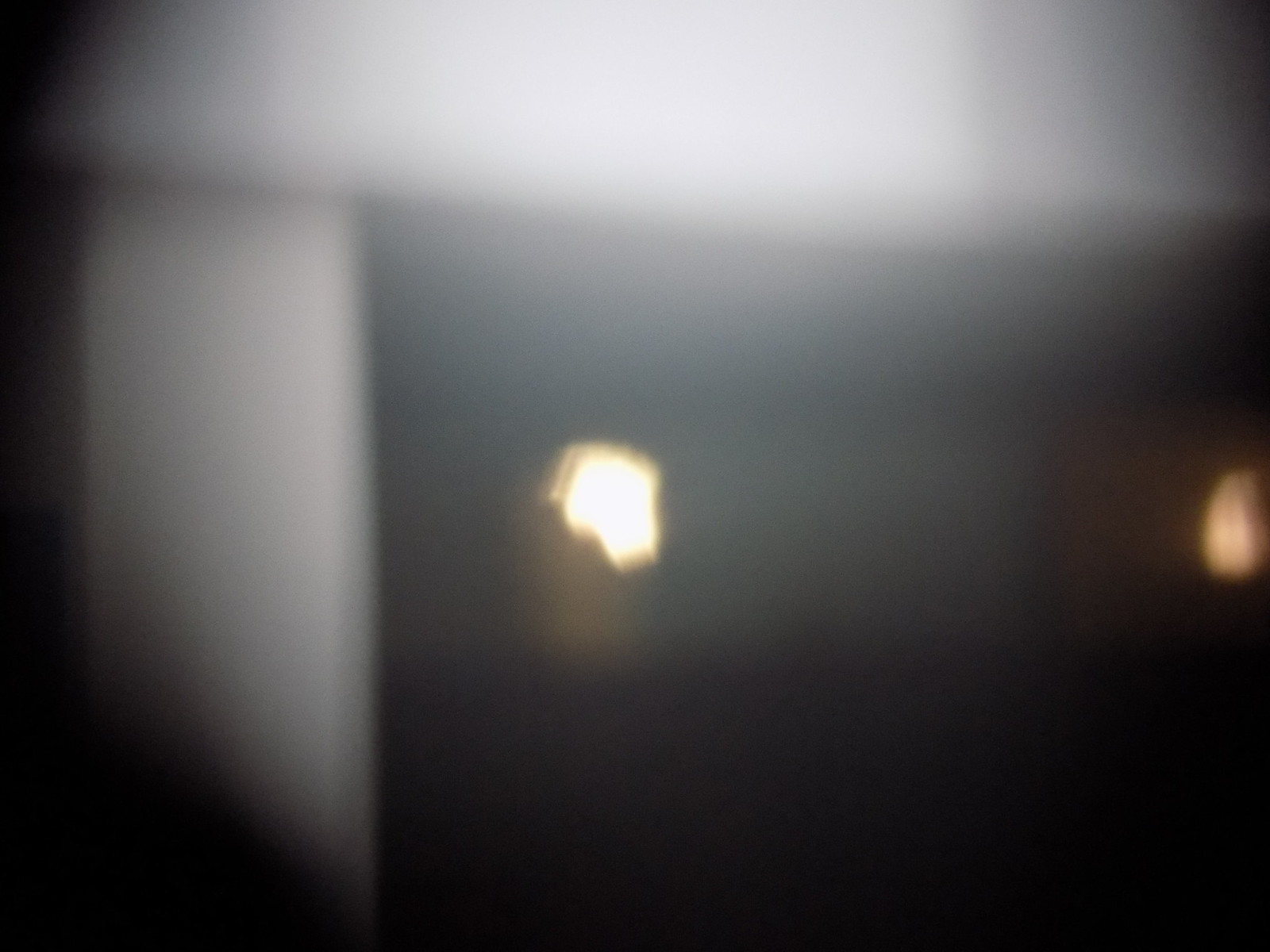This is a highly blurry and hazy image. The composition reveals a predominantly white left wall and ceiling, resembling the structure of a tent. Amidst the obscured backdrop, there are two distinct yellowish areas positioned symmetrically on the left and right sides, reminiscent of small, fiery orbs. The background possibly hints at another white wall, although it's faintly visible. The bottom portion of the image showcases a dark floor. No discernible objects can be identified due to the blurriness.